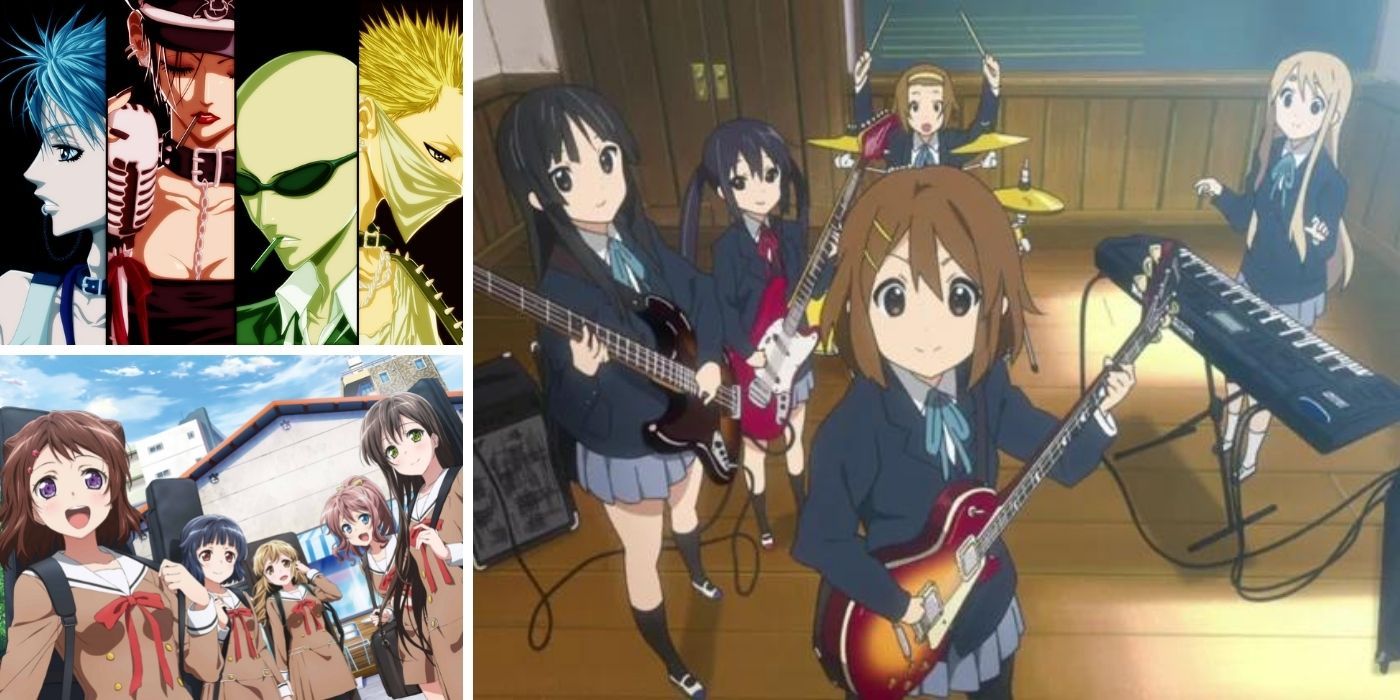The rectangular image, approximately 5 inches wide and 2 to 3 inches high, is divided into three distinct sections. The left section is subdivided into two smaller parts by a thin horizontal white line. In the upper left corner, there are four distinct anime characters: one with blue hair, another with red hair standing before a microphone, a bald man in green with sunglasses and a cigarette, and a masked character with spiky yellow hair. Directly below, five schoolgirls in brown uniforms are seen standing outside, smiling. Each girl has distinct hair colors including brown, black, blonde, red, and another shade of brown. The right section of the image shows the same schoolgirls now playing musical instruments in a classroom while dressed in dark gray uniforms. The scene includes a drummer in the background, three guitarists on the left, and a blonde girl playing keyboards on the right. The tall buildings in the background of the outdoor scene suggest a less urban Japanese city setting.